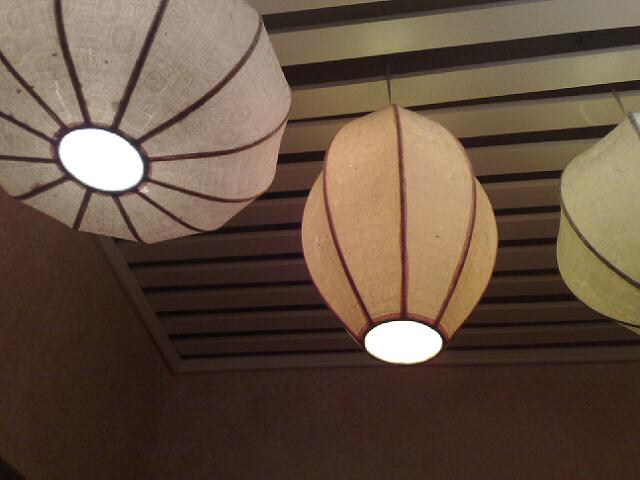This close-up image captures three paper lanterns hanging from a lightly colored, wooden-indented ceiling. The lanterns have distinct shapes; the one on the left is round and gray with dark horizontal lines, while the one in the middle is more oblong and pinkish with darker pink lines. Partially visible on the right, the third lantern is green with dark green lines and is cut off by the edge of the frame. Each lantern has a round opening at the bottom that allows light to shine through, illuminating the somewhat dark bottom portion of the image. They are all suspended from the ceiling via metal grates, emphasizing their traditional yet varied styles.